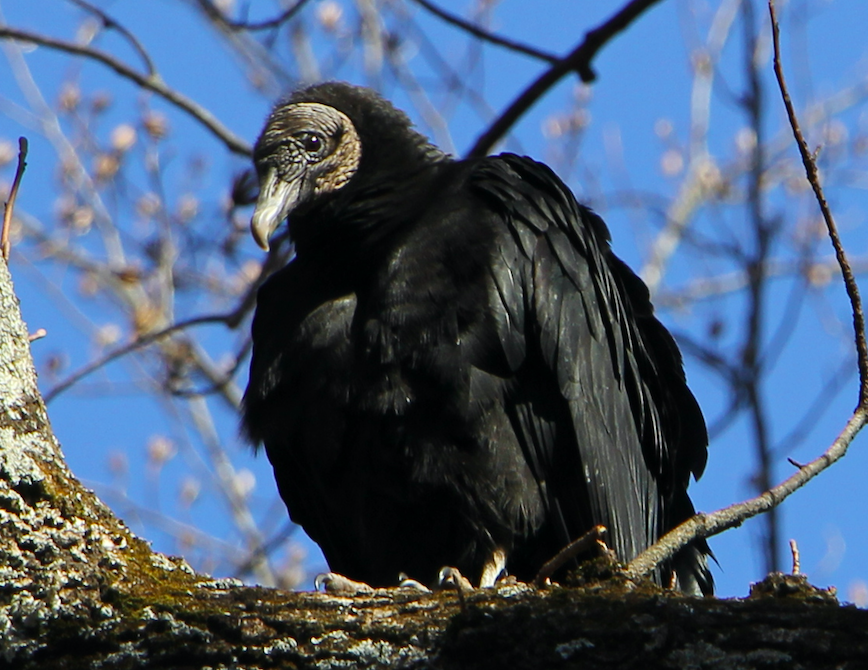The image showcases a large black vulture perched on a tree branch. The bird, with its body covered in large black feathers, has a wrinkly, featherless head that is a lighter gray color, reminiscent of a turkey. Its sharp talons, also grayish in color, grip the branch tightly. The vulture's beady black eye and long gray beak stand out prominently. The tree branch, extending horizontally and speckled with white, bears moss and gives the appearance of an oak tree. The background features a blue sky with blurry tree branches and brown foliage, indicating that the photograph is taken from a low angle looking upwards. The vulture, facing slightly to the left, appears vigilant as it sits still, framed by the natural surroundings.